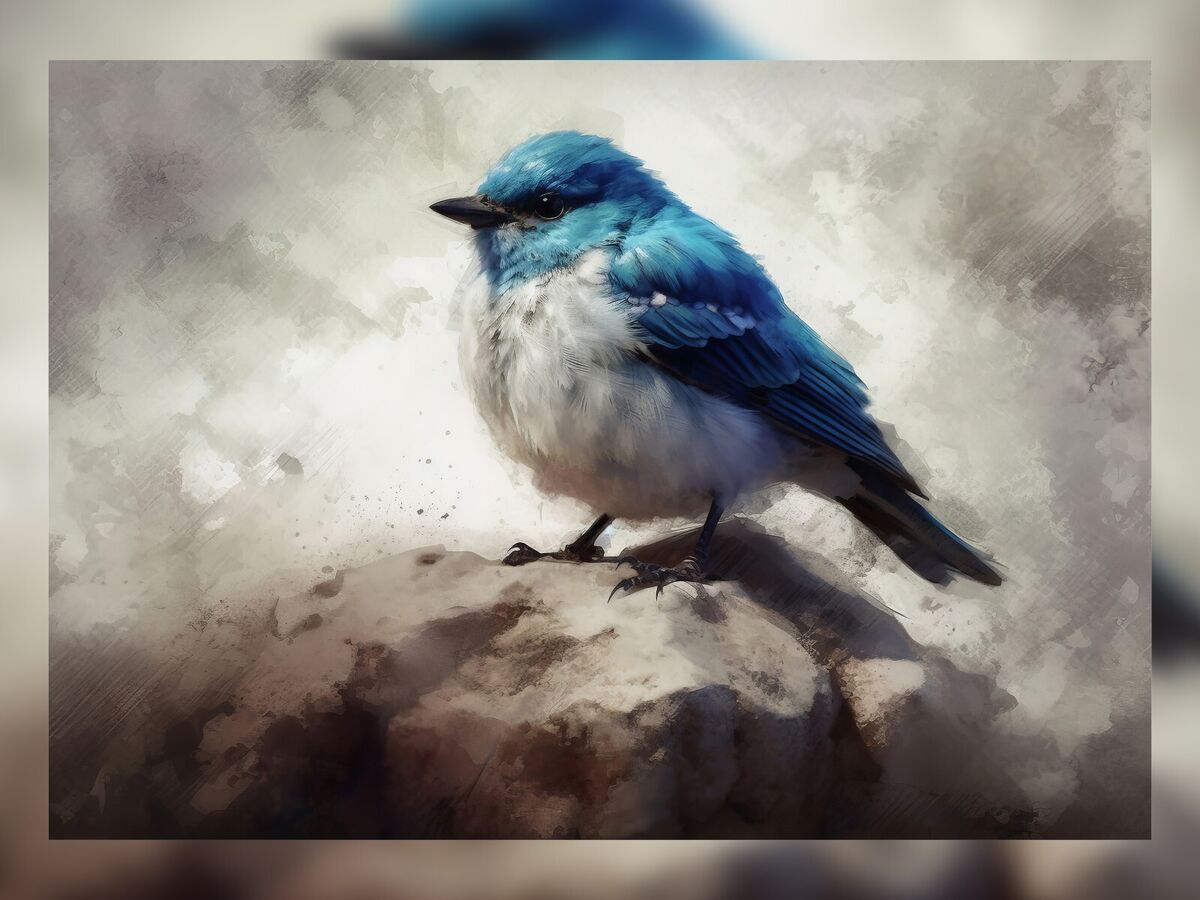This detailed image appears to be a hand-drawn or digitally crafted piece of art, featuring a central blue bird with a notably thick, fluffy body. The bird's head, wings, and part of its tail feathers are a striking blue, contrasting with its white underbody. Its legs, beak, and eyes are depicted in dark hues, adding to the bird's distinct features. The bird is perched on a tan-brown, bumpy rock that spans the width of the artwork's lower section. The scene is set against a less detailed, sketch-styled background in shades of grey with wave-like motions, enhancing the bird’s prominence. Interestingly, the entire scene is framed by a blurred, zoomed-in version of the main image itself, slightly visible towards the edges. The bird is centrally positioned, looking left, with its head nearly touching the top, making it the undeniable focal point of this beautifully intricate painting.